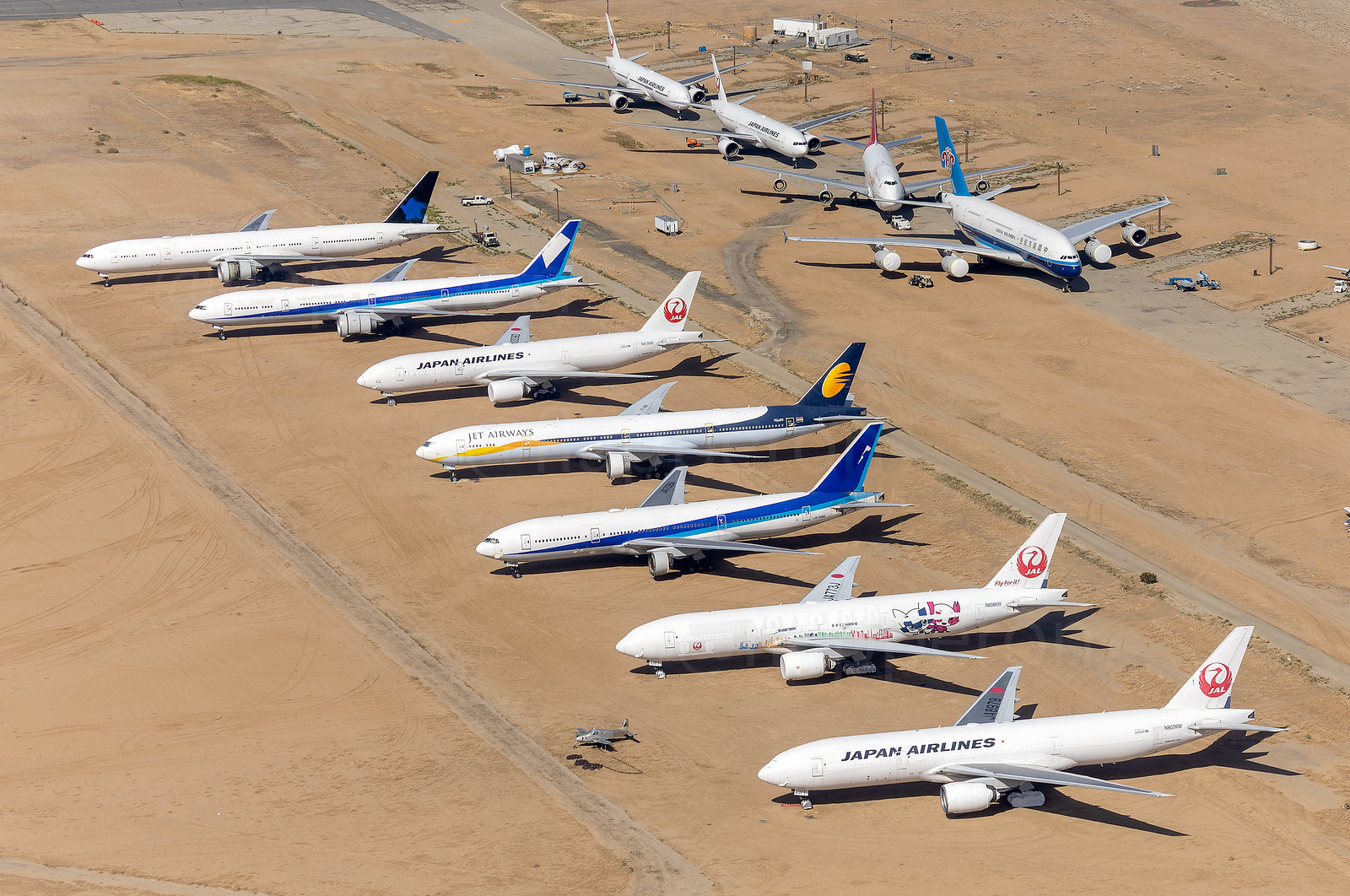This aerial photograph captures an outdoor scene within a desert landscape, depicting approximately 11 commercial jets in excellent condition. Most of the aircraft, which appear to be Boeing 767s, are predominantly white with some bearing colored stripes along their sides. Several planes are from Japan Airlines, while others have indistinct logos, likely from various Asian airlines, including one labeled Jet Airways. 

The planes are positioned on a dirt surface interspersed with service roads. Seven of the jets are aligned side-by-side facing west, parked closely together, indicating they are not preparing for takeoff. Meanwhile, four jets are lined up one behind the other, facing south, also parked. Vehicles can be seen around these planes, suggesting that this area may serve as either a maintenance site or a storage location for these aircraft. The photograph, taken from an altitude of about 400 to 500 feet, offers a clear view of this potential plane graveyard, though the jets themselves appear well-maintained.